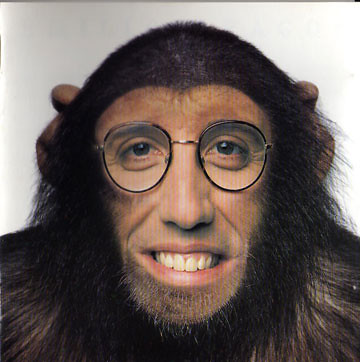The image depicts a surreal, digitally altered chimpanzee with an amalgamation of human facial features and elements. The chimpanzee's body and head are covered in typical brown hair, with large ears positioned towards the back, reflecting its natural appearance. However, the face is strikingly human, featuring brown eyes adorned with round, black-rimmed glasses, and a human nose and lips. The glasses have a metal bridge that spans across the nose. The human-like face displays a smile, revealing regular human teeth. This bizarre hybrid is set against a plain white background, emphasizing the stark contrast between the human and animal characteristics.